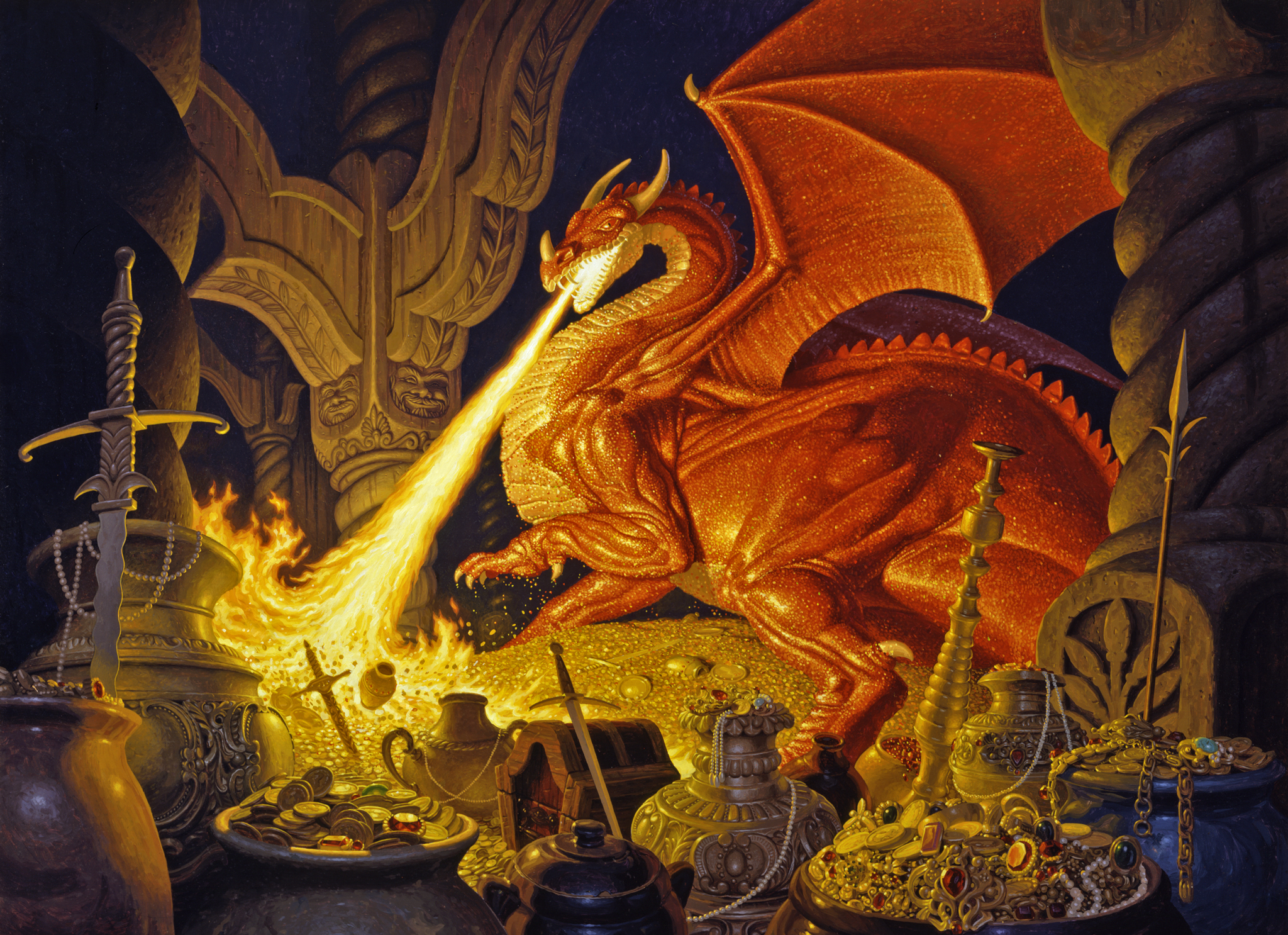The image is a detailed illustration of a menacing red dragon, reminiscent of Smaug from J.R.R. Tolkien's "The Hobbit," located in a dark, vault-like chamber. The dragon, with its muscular legs and prominent horns—two large ones on its head and a smaller one jutting from its nose—dominates the scene. Its head is angled towards the ground, mouth open wide as it breathes fire onto a lavish hoard of treasure. The dragon's outstretched wings enhance its imposing presence. Surrounding the dragon and scattered in the foreground are treasures from its hoard, including gold coins, jewelry, an ornate chest, a large spear, swords, urns, a candlestick, and various other luxurious items. The dragon stands atop a pile of gold, and the chamber itself is supported by intricately carved wooden shafts, adding a touch of craftsmanship to this fantasy setting. The glow from the dragon's fire illuminates the otherwise dark chamber, emphasizing the dragon’s fierce guardianship over its amassed wealth.